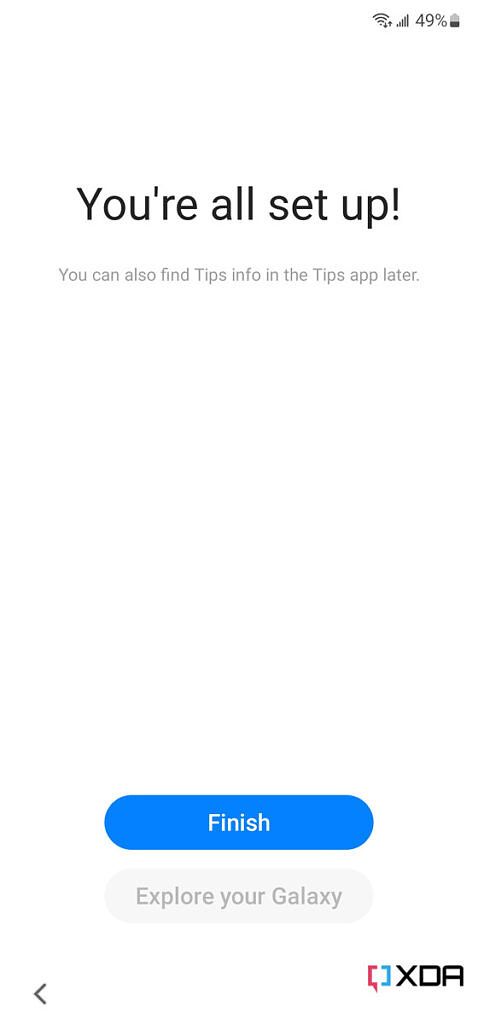This image is a screenshot of a completion screen on a Galaxy Android device. The entire page has a clean white background. At the top, the status bar displays the Wi-Fi strength, signal strength, and a battery icon showing 49% charge.

Central to the image is large, bold black text stating, "You're all set up!" Beneath this message, smaller gray text reads, "You can also find tips info in the tips app later."

The page features considerable white space for a minimalist look. Near the bottom, a prominent blue oval button with white letters says, "Finish," and adjacent to it is another oval button in gray with the text, "Explore your Galaxy."

The bottom-left corner features a left-pointing arrowhead, indicating a possible navigational option. On the bottom-right, red and blue brackets face each other, enclosing the black letters "XDA," presumably indicating a connection to the XDA Developers community or resources.